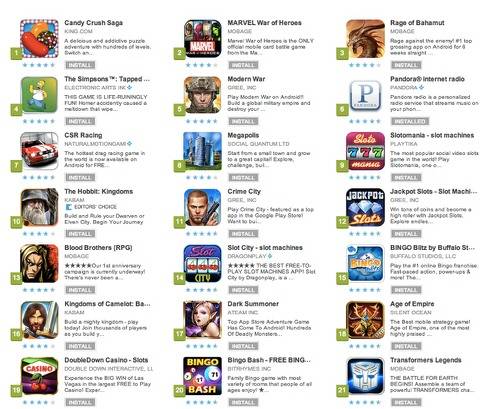This image is a screenshot of the mobile app store, specifically the Play Store, showcasing a ranked list of the top 21 games. The layout consists of three columns and seven rows, displaying a total of 21 games. Each game is represented with a colorful icon and includes essential information such as the game's name, developer, a brief description, and its ranking, which is indicated by a green square in the bottom-left corner of each game's section.

- **Rank 1: Candy Crush**
  - **Developer:** King
  - **Description:** Delicious and addictive puzzle adventure with hundreds of levels.
  - **Icon:** Features candy items.

- **Rank 2: Marvel War of Heroes**
  - **Developer:** Rage of Belmont
  - **Description:** Engaging superhero card battle game.

- **Rank 3: The Simpsons: Tapped Out**
  - **Developer:** EA Mobile
  - **Description:** Build your own Springfield in this city-building game.

- **Ranks 4-21:**
  - **Modern War**
    - Developer: Funzio Games, Inc.
    - Description: Conquer the world in this military strategy game.
  - **Pandora Radio**
    - Developer: Pandora
    - Description: Personalized music and radio streaming service.
  - **CSR Racing**
    - Developer: NaturalMotionGames Ltd
    - Description: High-stakes drag racing game.
  - **Megapolis**
    - Developer: Social Quantum Ltd
    - Description: City-building strategy game.
  - **Slotomania**
    - Developer: Playtika
    - Description: Free slots casino game.
  - **The Hobbit: Kingdoms**
    - Developer: Kabam
    - Description: Strategy game based on "The Hobbit" movie.
  - **Crime City**
    - Developer: Funzio Games, Inc.
    - Description: Crime-themed strategic RPG.
  - **Jackpot Slots**
    - Developer: Phantom EFX
    - Description: Vegas-style slot machine game.
  - **Blood Brothers**
    - Developer: DeNA Corp.
    - Description: Dark fantasy RPG.
  - **Slot City**
    - Developer: GameHouse
    - Description: Casino slot machine game.
  - **Bingo Blitz**
    - Developer: Playtika
    - Description: Free multiplayer bingo game.
  - **Kingdoms of Camelot**
    - Developer: Kabam
    - Description: Medieval empire-building game.
  - **Dark Summoner**
    - Developer: Ateam Inc.
    - Description: Monster battle RPG.
  - **Age of Vampire**
    - Developer: Good Game Studios
    - Description: Action-packed RPG.
  - **Double Down Casino Slots**
    - Developer: Double Down Interactive LLC
    - Description: Casino game with various slot machines.
  - **Bingo Bash**
    - Developer: GSN Games, Inc.
    - Description: Fast-paced bingo game.
  - **Transformer Legends**
    - Developer: DeNA Corp.
    - Description: Card battle game featuring Transformers.

Each game is depicted with vibrant, full-color graphics, making the list visually appealing and easy to navigate for users looking to explore popular game options.